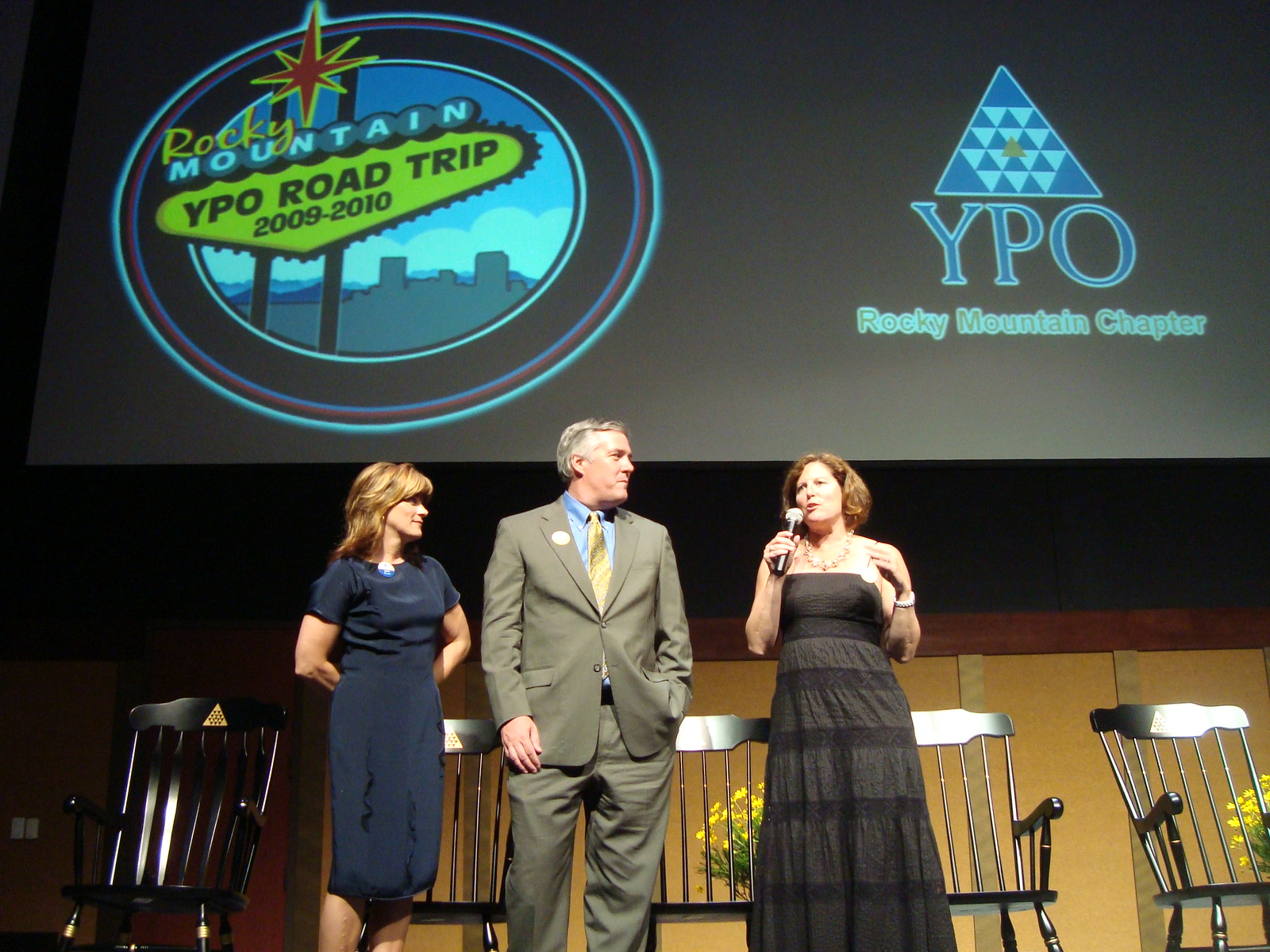In this photograph, three individuals are positioned on a stage, set against a backdrop featuring five black chairs that resemble rocking chairs and a vibrant projection screen. The woman on the far left is dressed in a navy blue dress with short sleeves, extending just below her knees, and her hands are held behind her back as she faces the other two individuals to her right. The central figure is an older Caucasian man with gray hair, dressed in a light gray suit paired with a blue shirt and gold tie. He stands confidently with one hand in his pocket and the other positioned near his hip. The woman on the far right, also Caucasian, sports a black dress and holds a black microphone to her partially open mouth, as if in mid-speech. She has short red hair that falls just below her ears and wears a necklace adorned with pink trinkets. Behind the trio, there are chairs decorated with a yellow triangle on the leftmost one, and arranged behind them are green flowers topped with blue blooms. Above them, the banner spanning the top of the image is marked with two emblems: on the left, a circle with a red star encircled by the text "Rocky Mountain YPL Road Trip 2009-2010," and on the right, a blue triangle with inner light blue and green triangles, accompanied by the text "YPL Rocky Mountain Chapter." This image captures a moment during what appears to be a presentation or speech at an event.